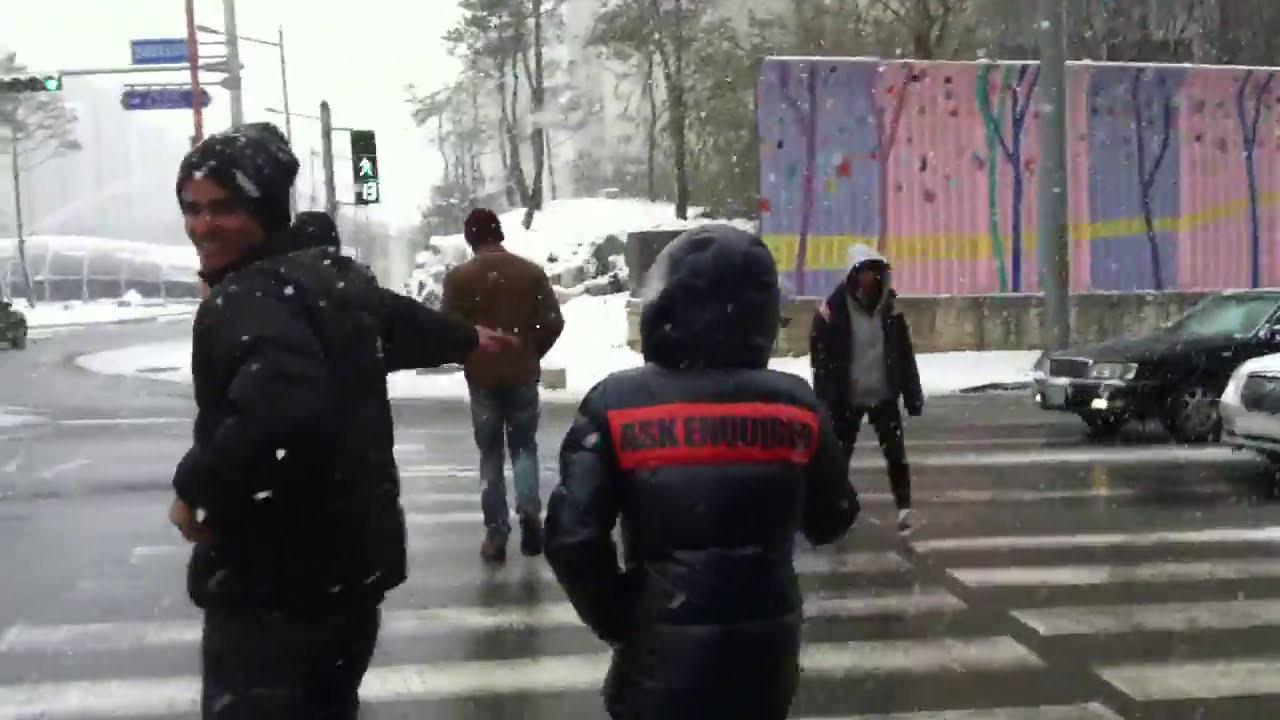The image captures a bustling city intersection in the midst of winter. The green pedestrian signal is illuminated, showing a walking figure and the number 13, indicating the seconds left to cross. Four men are visible at the crosswalk: three are walking forward, one in a black coat glances back over his left shoulder, his dark skin and features contrasting with the snow. Another man in a black coat with a red stripe and some unreadable black text on it points his forearm across the crosswalk. The two other men in the foreground wear a brown coat with jeans and a gray hoodie under a black coat, respectively, while the man walking in the opposite direction also braves the cold. Snow lightly falls, dusting the ground and creating small patches alongside the roads. On the side, a white car and a black car wait patiently for the pedestrians to pass. Street signs, road markings, and dotted lines guide the way. In the background, a city mural adorned with vibrant colors—purple, pink, yellow—depicts simple tree shapes, giving a touch of artistic flair to the urban landscape. Nearby, trees laden with snow hint at a park or woodland area beyond the intersection, adding a natural element to the wintry scene. The roads are relatively clear, but snow blankets the sidewalks and treetops, emphasizing the season's presence.